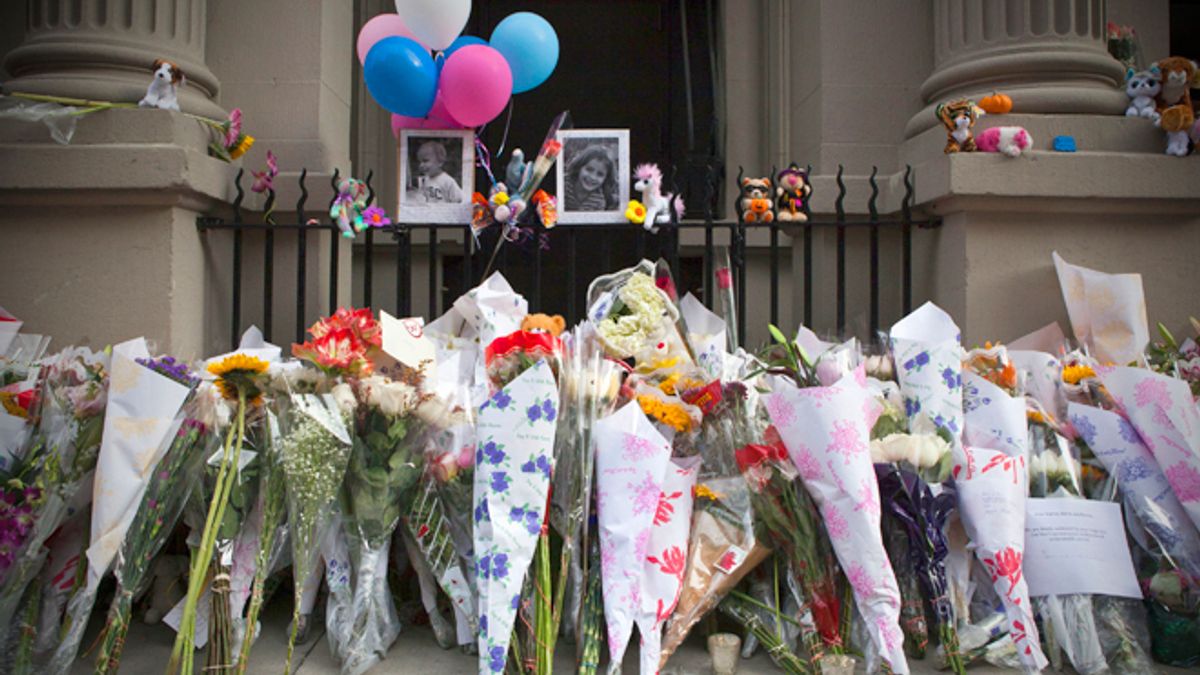The image depicts a poignant memorial set against a beige building with a black wrought iron gate. The memorial features numerous unique bouquets of flowers, each distinct with various colors including white, red, and orange, all neatly arranged and leaning against the gate. Above the flower arrangements, there are two black-and-white photographs: one of a baby and another of a slightly older child, possibly around six years old with shoulder-length hair. Tied near these photos are an assortment of balloons in pink, blue, and white. Additionally, scattered along the gate and at the base of the memorial are various stuffed animals, including teddy bears and toy puppies, some of which are placed on the lower parts of the metal fencing and atop the columns flanking the gate. The overall scene suggests a heartfelt tribute to the memories of the children, with each element contributing to the somber yet touching atmosphere.